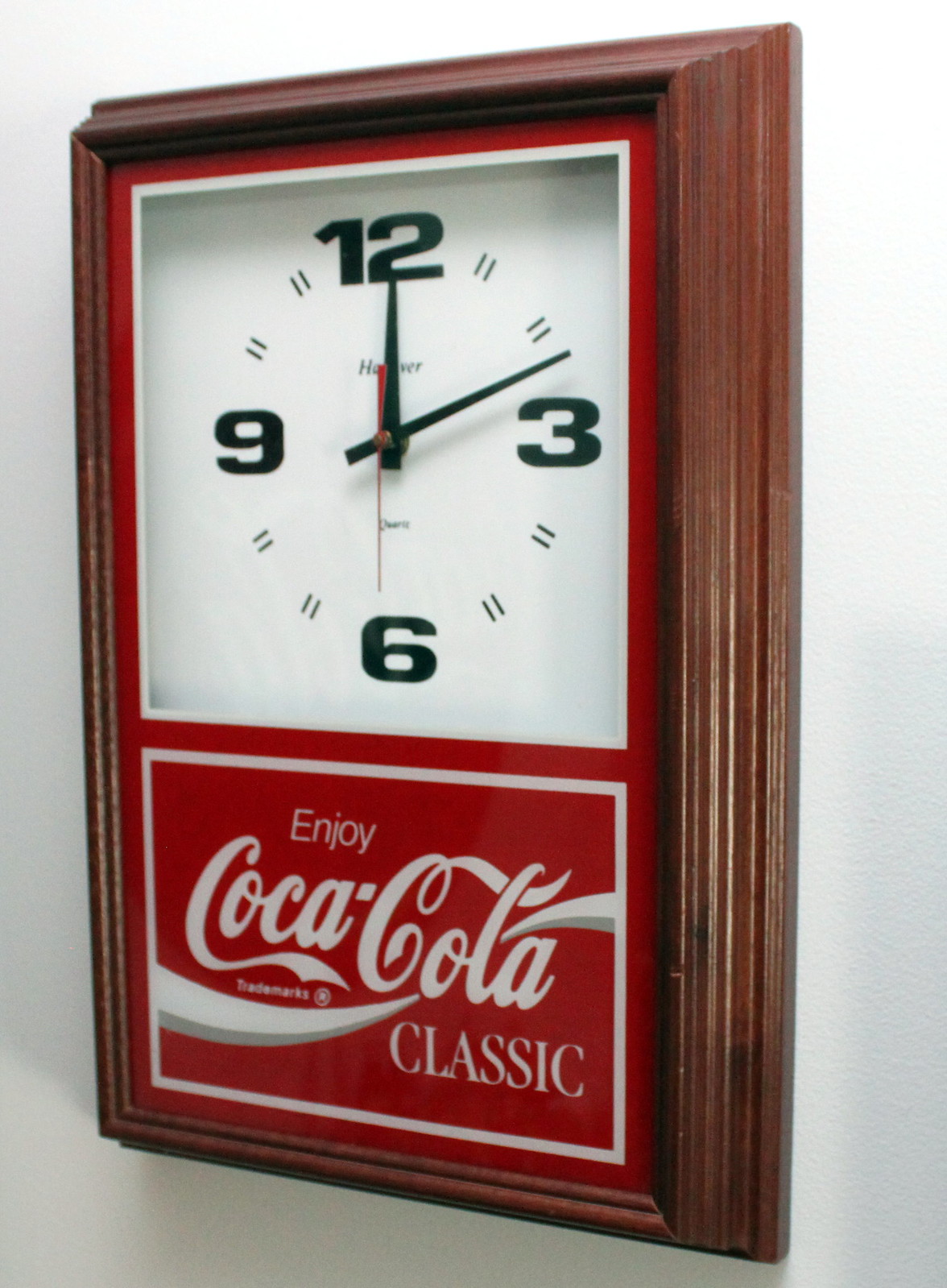A vintage Coca-Cola wall clock is prominently displayed against a background. The clock is enclosed in an ornate, dark brown wood frame with intricate ridges that could easily gather dust, adding to its rustic charm. The distinctive clock face occupies the upper two-thirds of the design and features black numerals with elegant clock hands set at 12:12. Partially obscured by the hands, the name of the manufacturer, possibly "Hanover," can be faintly seen. Below the clock face, a vibrant rectangular panel occupies the bottom third, adorned with the iconic Coca-Cola Classic slogan in white text on a bold red background, bordered by a contrasting white edge. This nostalgic timepiece merges classic advertising with timeless functionality.